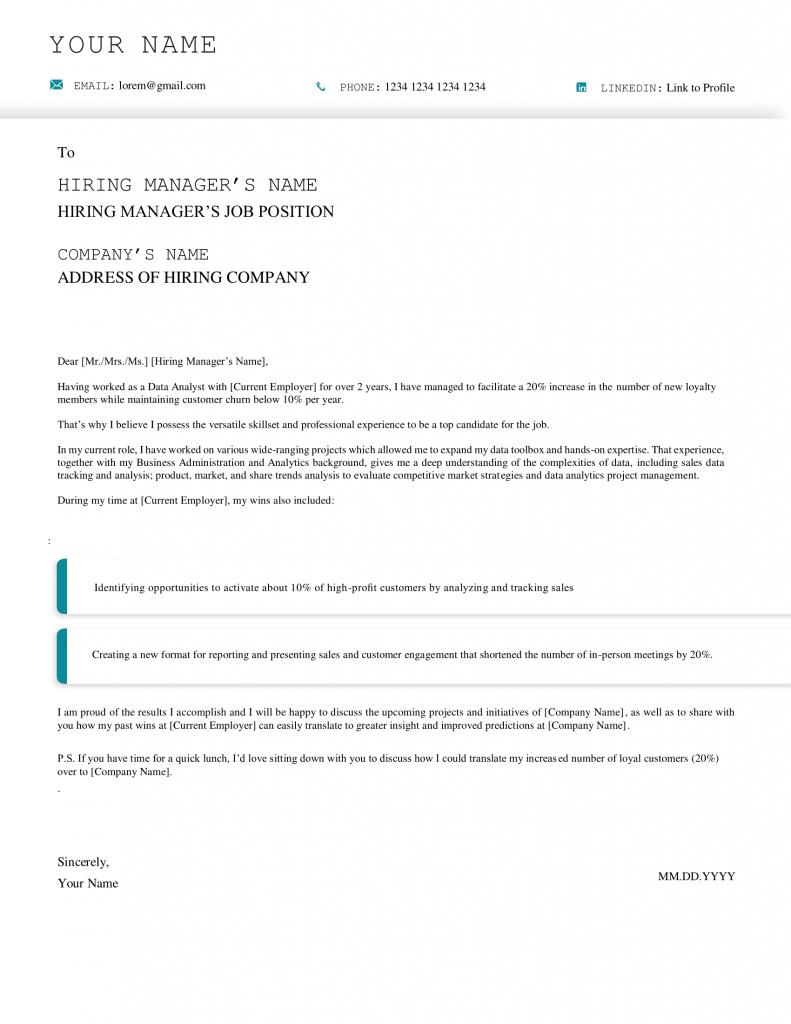**Detailed Caption:**

A typewritten form letter aimed at applying for a Data Analyst position is displayed. At the top, it starts with a placeholder for the applicant's name, followed by the email address "iorem@gmail.com," a placeholder phone number "123-412-34," and a LinkedIn profile link. 

The letter is addressed to "Hiring Manager's Name," "Hiring Manager," "Job Position," at "Company Name" with the company's address beneath. 

The salutation reads, "Dear Mr./Mrs./Ms. Hiring Manager's Name." The body of the letter begins by introducing the applicant's current role as a Data Analyst, mentioning a tenure of over two years. The applicant boasts facilitating a 20% increase in new royal members while keeping the customer churn rate below 10% per year. It highlights the applicant's versatile skills and professional experience, positioning them as a top candidate for the job.

A highlighted section of the letter emphasizes a key achievement: "Identified opportunities to activate about 10% of high-quality customers through the analysis of tracking sales." The section is visually marked with two bars having blue edges, drawing attention to this noteworthy accomplishment.